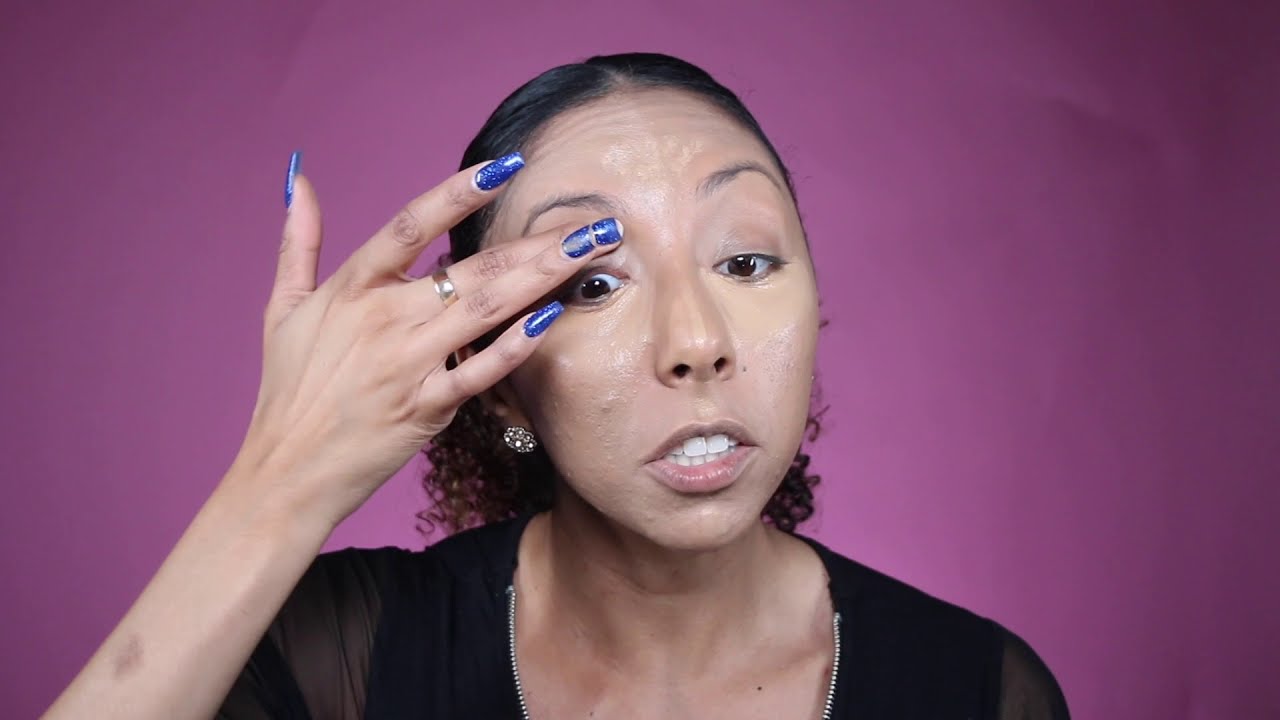In the image, a woman stands against a rich purple background that radiates from light to dark shades. She is depicted from the mid-shoulder up, wearing a thin black blouse featuring a zipper. The woman has black hair styled into a ponytail, exposing curls just below her neck. With her mouth slightly open, revealing her teeth as if saying a “ch” sound, she’s touching her right eyelid with her middle finger, pulling it up to reveal more of the white of her eye—possibly mimicking the action of putting in or taking out a contact lens. Her middle finger, adorned with a gold band, bears blue nail polish, though the nail is broken and shorter than the others. The fingernails appear to have a star design. Notably, she has diamond earrings and brown eyes, and her complexion reveals traces of acne scarring. The overall setting and her gesture suggest she might be applying or removing makeup near her eyebrow.